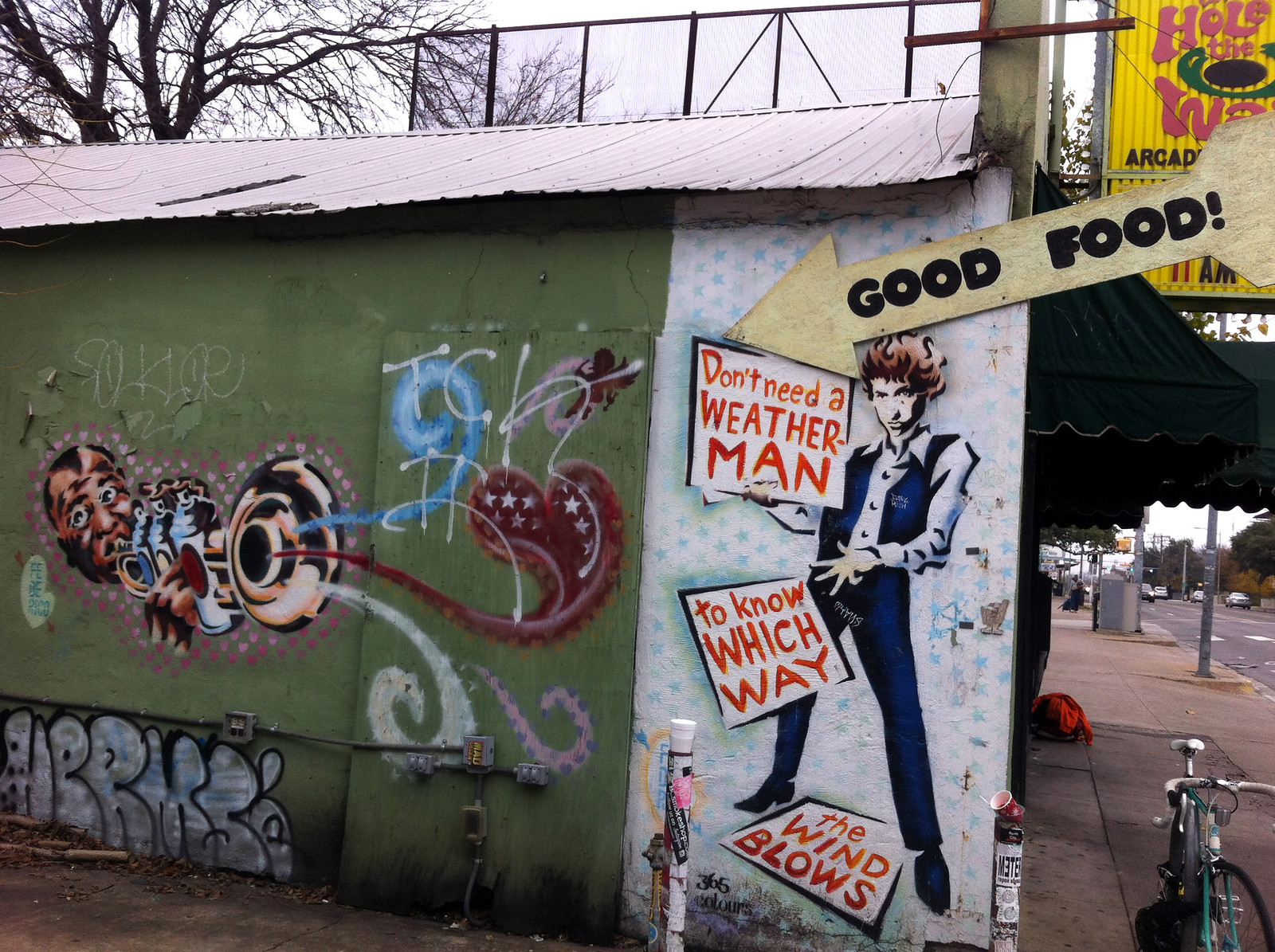The photograph is taken outside on a cloudy, overcast day, likely during late fall or winter, as the trees are bare and devoid of leaves. The scene is set along a road with a sidewalk, and features a store on the right-hand side. The store's wall, viewable from what appears to be an alleyway or the back of the store, is adorned with vibrant graffiti.

On the left side of the wall is a mural set against a brown or green background, depicting a black man playing a gold trumpet, the buttons of which are replaced by spray cans of paint. Colorful swirls—blue, white, pink, and red, the latter forming a heart—emerge from the trumpet's bell. 

To the right, the wall transitions to a white section patterned with blue stars or polka dots. Here, a caricature of a man with flaming hair is dressed in a blue vest and pants, and a white button-down shirt. He holds a sign that reads, "Don't need a weatherman to know which way the wind blows." An arrow at the top right of the wall points toward the store, proclaiming "Good Food" in black lettering.